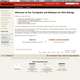This image is a blurry screenshot, potentially from a website or software interface. The top part of the image features a prominent red bar, although its contents are indistinguishable. Below the red bar, there's likely a thinner black bar. The left side of the screenshot includes a beige sidebar with a series of list-style buttons, but the text on these buttons is unreadable. The main section consists of a large white column occupying the majority of the space, approximately four times wider than the sidebar. At the bottom of the screenshot, there is a beige footer.